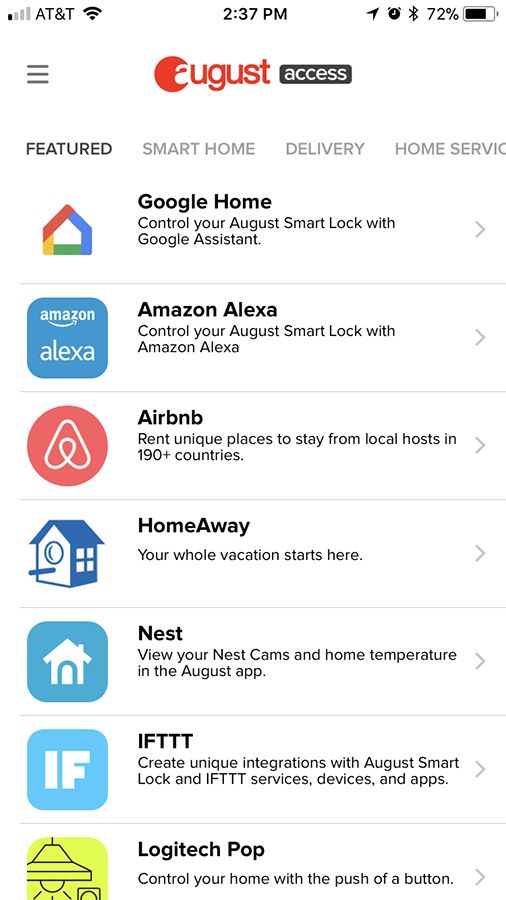The image depicts a screenshot of a cell phone, set against a solid white background. In the upper-left corner of the screen, one bar of reception is visible next to the "AT&T" label, with the Wi-Fi icon positioned to the right. At the center top of the screen, the time is displayed as 2:37 p.m. To the right of the time, several icons are visible, including an alarm clock and a battery indicator showing 72% charge.

Centered just below the top section, there is a black box containing the text "August access," with "August" in red and "access" in white. Underneath this heading, there is a list of apps. The first listing is "Google Home," accompanied by the Google Home icon on the left side. The text below this states, "Control your August smart lock with Google Assistant."

The second app in the list is "Amazon Alexa," which also comes with a brief description stating, "Control your August smart lock with Amazon Alexa."

The third app is "Airbnb," with the additional text, "Rent unique places to stay from local hosts in 190+ countries," providing a summary of the app's functionality.

Each element is presented clearly, making it easy to understand the functionalities and partnerships associated with August access.